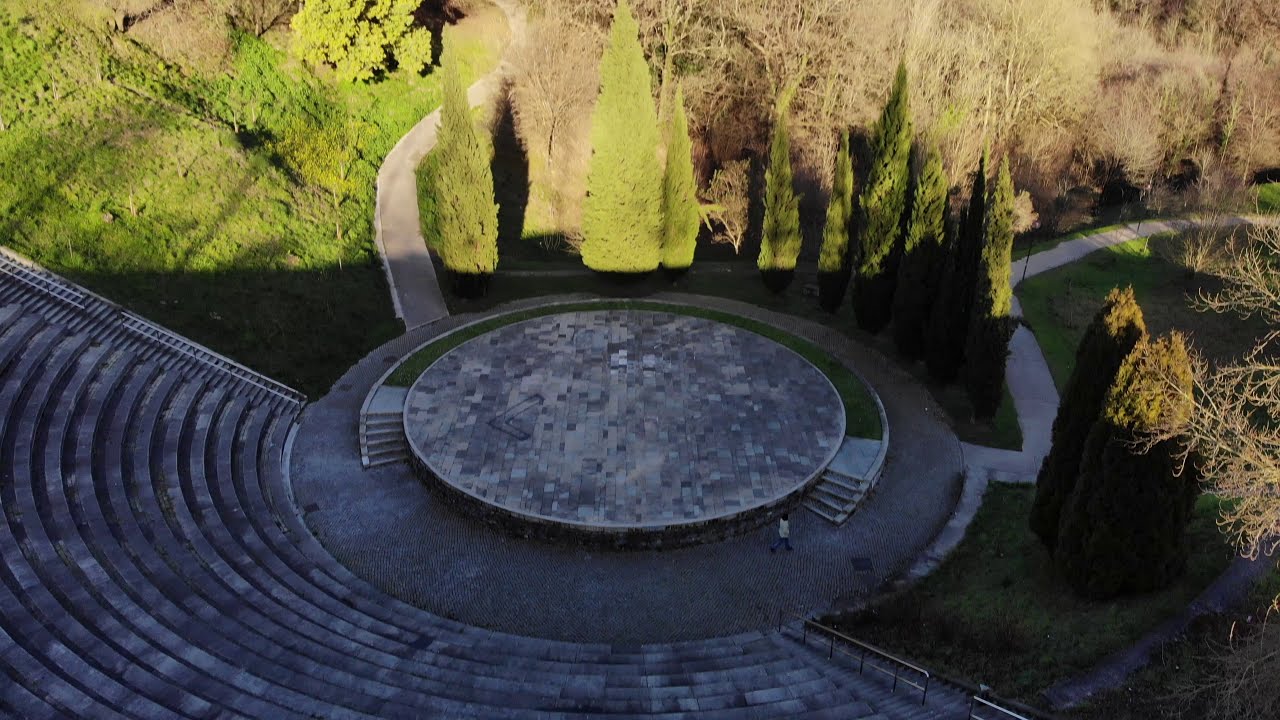This aerial photograph captures an outdoor amphitheater and stage set in a park, presented in a horizontal rectangular format. The central focus of the image is a circular stone stage with surrounding concrete bleachers arranged in a quadrant-like stadium seating on the left side of the stage. There are two pathways flanking either side of the stage, leading up to it.

The image, clearly taken from an elevated perspective on a relatively bright day, showcases a mix of deciduous and coniferous trees. In the background, deciduous trees can be seen without leaves, suggesting a winter setting, while tall pine or fir trees provide a lush, green backdrop that occupies around 25% of the stage area. The color palette is predominantly gray, green, brown, beige, black, and white.

The detailed composition suggests that this stage, possibly used for musical performances by local bands or orchestras, is reminiscent of an ancient ruin but is likely a contemporary structure designed for outdoor events. The shading across the stage and the seating areas add depth to the scene, enhancing the picturesque, postcard-like quality of the image.